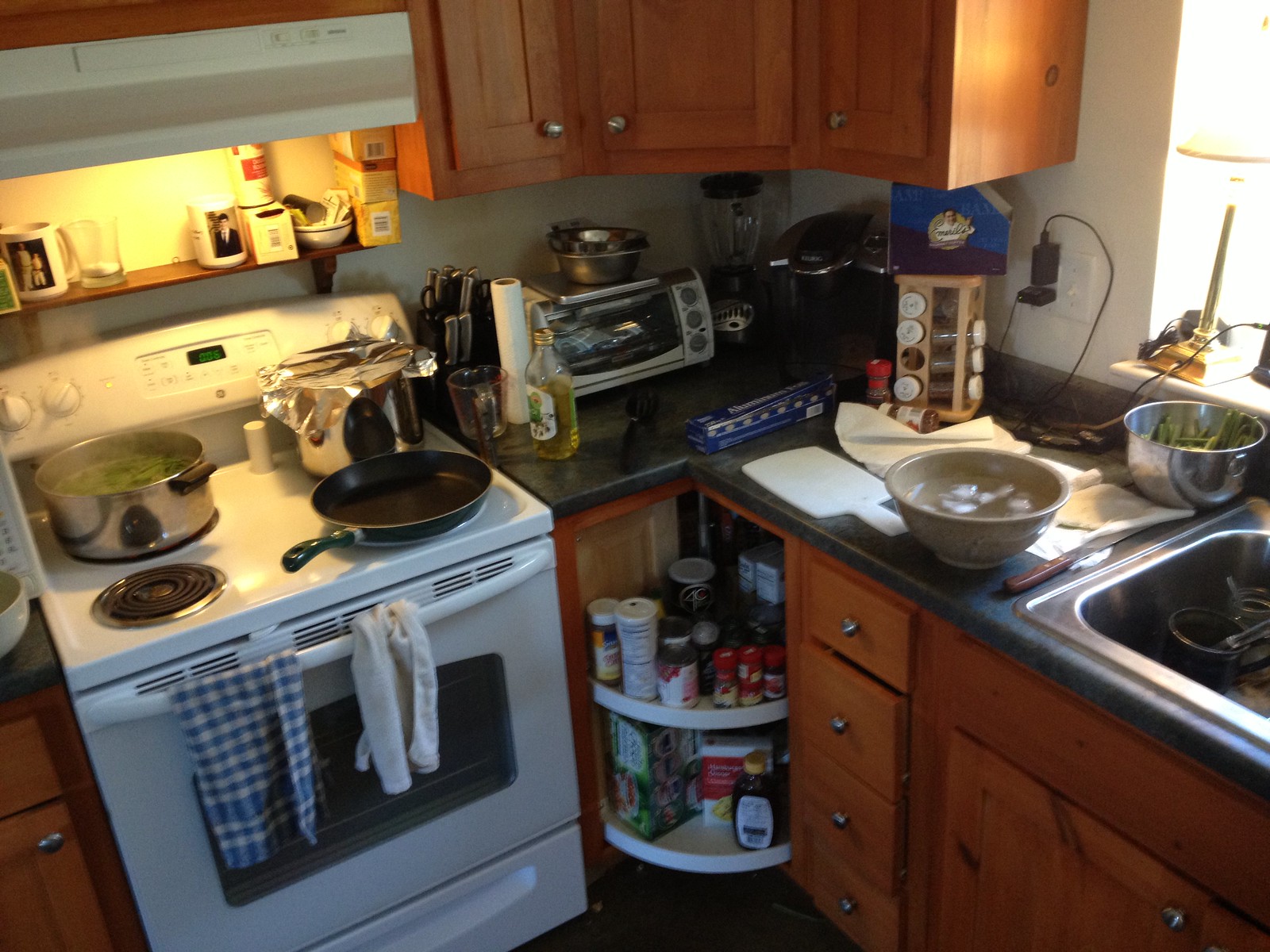The image depicts a well-used kitchen, with various cooking activities underway. On the top left of the stove, there is a pot of greens boiling down. Towards the bottom left, a pan is in use, possibly cooking another part of the meal. On the top right of the stove, there's another pot with tinfoil covering its top, perhaps to retain warmth or moisture.

In the corner of the kitchen counter, you can see a mini convection oven, alongside a blender and a K-cup coffee maker, indicating a busy and functional cooking space. There are two spice racks; one is visible on the countertop, while another corner spice rack is mounted below, offering a range of seasonings for diverse culinary creations. 

An empty bowl is also present, though its use is not clear from the picture. On the right side of the image, a container of string beans is waiting to be prepared or cooked.

Overall, this kitchen appears organized yet active, reflecting someone in the midst of meal preparation.